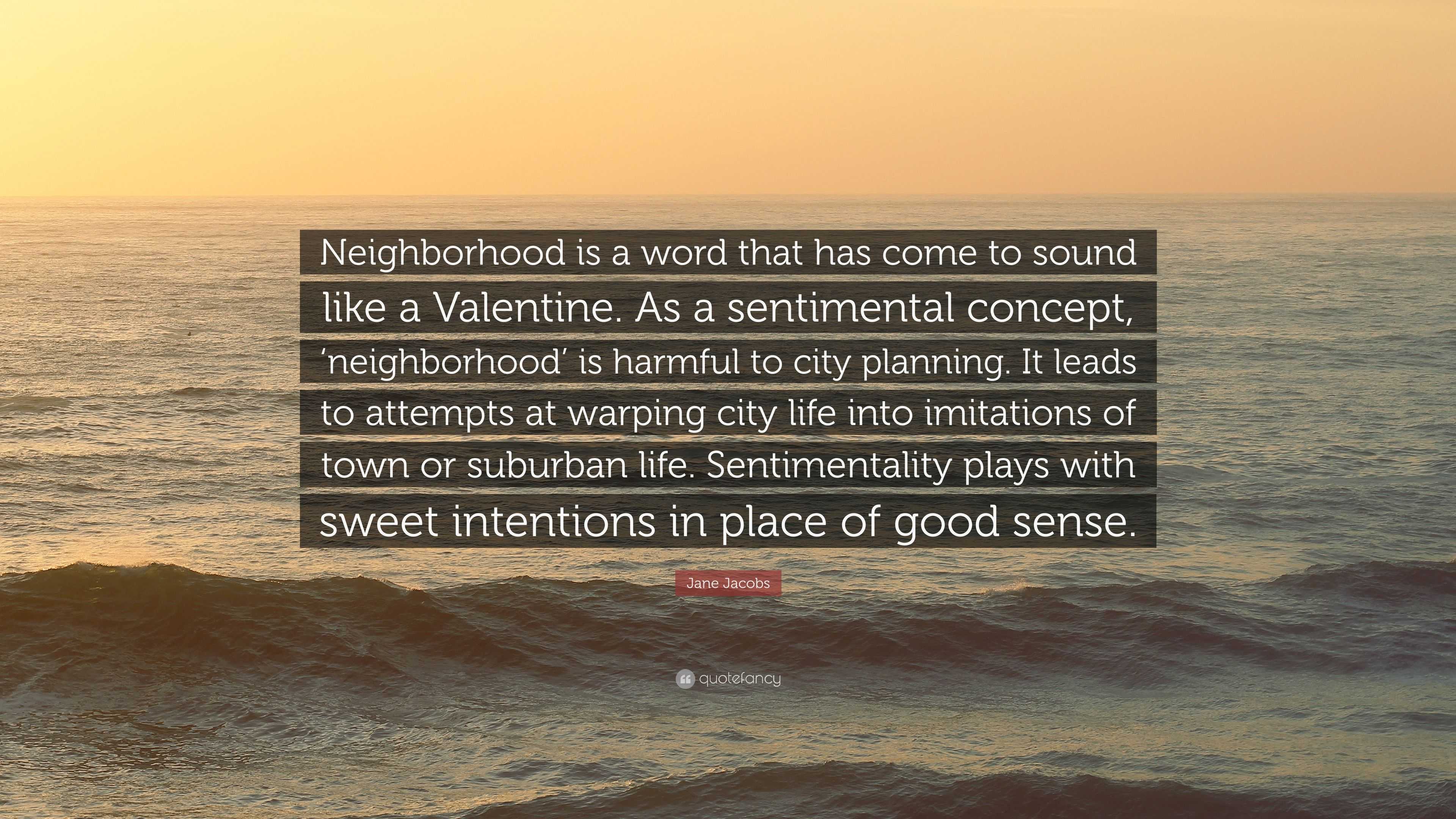The image depicts a serene body of water, possibly an ocean or lake, with gentle waves breaking towards the shore. The sky, an array of vibrant oranges and yellows, indicates the recent setting of the sun, casting a reflective glow on the dark blue water below. In the middle of the scene, a brown square with white text interrupts the natural beauty, carrying a rather perplexing message: "Neighborhood is a word that has come to sound like a valentine. As a sentimental concept, neighborhood is harmful to city planning. It leads to attempts at warping city life into limitations of town or suburban life. Sentimentality plays with sweet intentions in place of good sense." Below this text, a smaller red square declares the author, Jane Jacobs, though a mispronunciation renders her name as June in some interpretations. The overall image juxtaposes the tranquility of nature with a controversial statement about urban planning, creating an intriguing and thought-provoking visual experience.